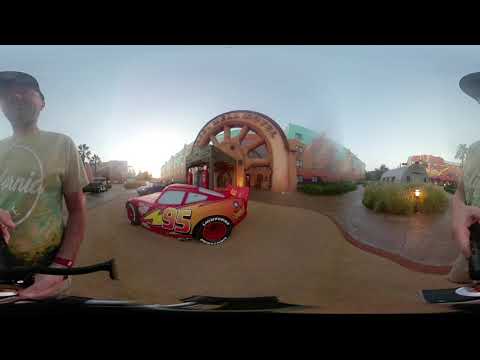In this outdoor 360-degree photo, a man stands in the left corner, blurred, wearing a green t-shirt with a white circle and partial text reading "NIC." He also has a red wristband and a black baseball cap. The centerpiece of the image is a sporty red and yellow race car, emblazoned with the number 95 and a yellow lightning bolt on its side. The car's windows are tinted white, and it has distinctive black wheels with red centers. Surrounding the car, there are various parked vehicles, including a black sporty car and a black van on the left side. The backdrop features a façade resembling a rusty-colored sun connected to a large archway, behind which stands a teal building. Additional red and yellow smaller buildings or possibly amusement rides, along with ground lights, are visible on the grassy right side. The sky is a clear, vibrant blue, without any clouds.